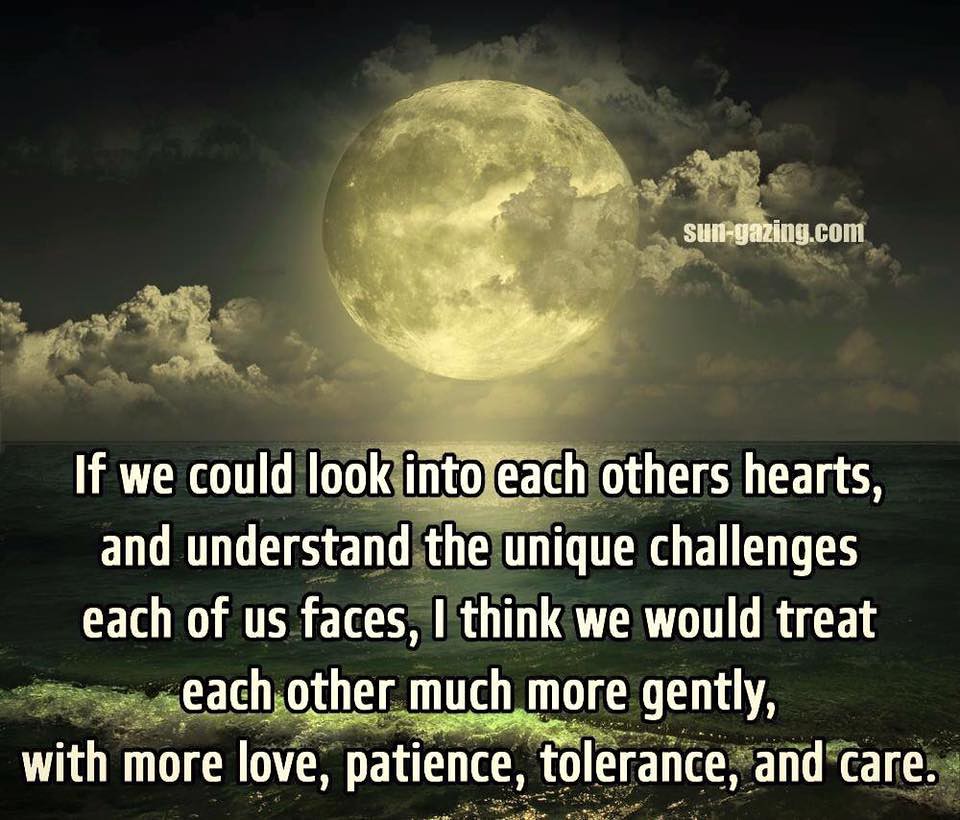The photograph is a square graphic depicting a tranquil night scene featuring a detailed image of a moon hanging over a vast body of water, likely a sea or ocean. The moon is positioned in a darkish blue sky, partially veiled by clouds on either side, and its reflection shimmers on the water's surface, accentuating the serene atmosphere. Below the moon, white text gracefully overlays the water, stating: "If we could look into each other's hearts, and understand the unique challenges each of us faces, I think we would treat each other much more gently, with more love, patience, tolerance, and care." This thoughtful and heartfelt message is presented in a nice, bubbly font. At the bottom of the image, a bit of the shoreline is visible, anchoring the ethereal scene to a tangible location. The photograph also subtly includes the website sungazing.com, indicating its origin.